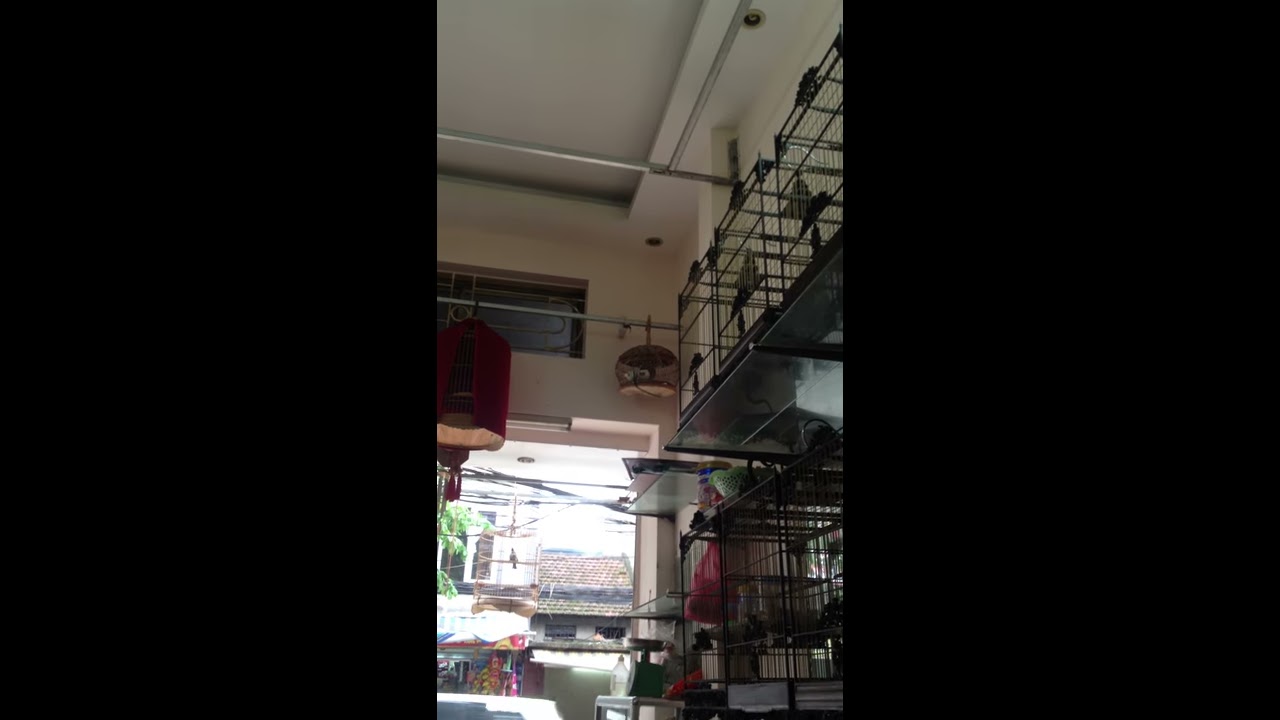The image captures the interior of a garage-like building that serves as part of an open-air market, possibly in an Asian setting. The scene is framed vertically by black bars on either side, emphasizing the tall, narrow perspective. The building's walls and ceiling are painted in white and ivory tones, and there are various birdcages arranged within the space. On the right wall, five tall, rectangular black birdcages are visible, adorned with assorted items such as fruit bowls and canisters.

Above the open front entrance, which looks out onto a street with another square garage-like building, hangs a silver pole with two birdcages. The left cage on the pole is an antique-looking, round design covered with a red velvet curtain, while the cage to its right is smaller, squat, and currently empty. The view through the entrance reveals utility lines crossing the top and a partly visible rooftop against an overexposed sky.

In addition, a cutout portion of the ceiling features two recessed can lights and a bar system. Adding to the vibrant market atmosphere, decorative red paper lights hang down from the ceiling, and cable lines are visible at the top of the doorway. The lower part of the image hints at a bustling market environment outside, with tented areas for vendors to display their goods, suggesting a lively and functional space.